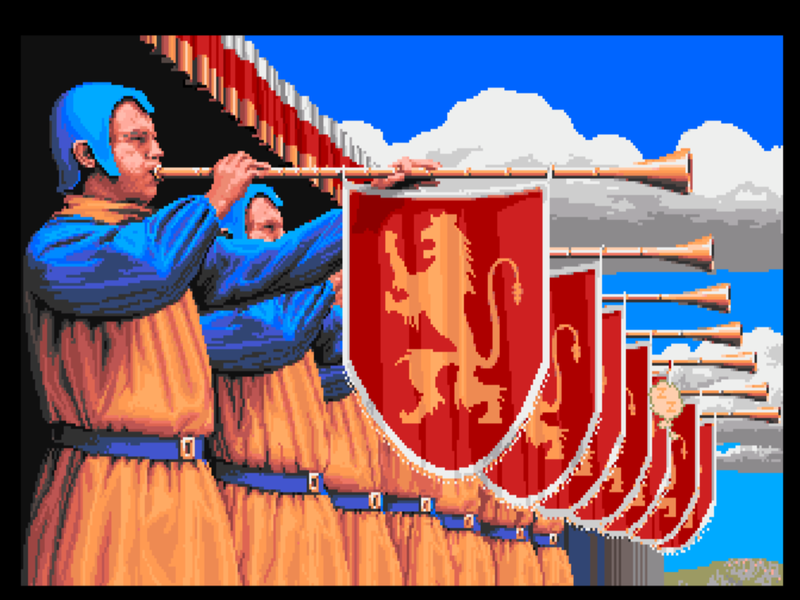The image depicts a pixelated, computer-generated scene reminiscent of a medieval ceremony. A row of seven men stands with only the first two faces visible, each dressed in tangerine-colored tunics with royal blue belts, sleeves, and caps. They hold long trumpets from which red and white banners hang, each adorned with a tangerine-colored lion rearing up on its hind legs. The background features a bright blue sky with puffy, cartoon-like white clouds. Above the men's heads is a border of the structure they're in front of, characterized by white, red, and orange colors. The overall atmosphere suggests an announcement or celebration.